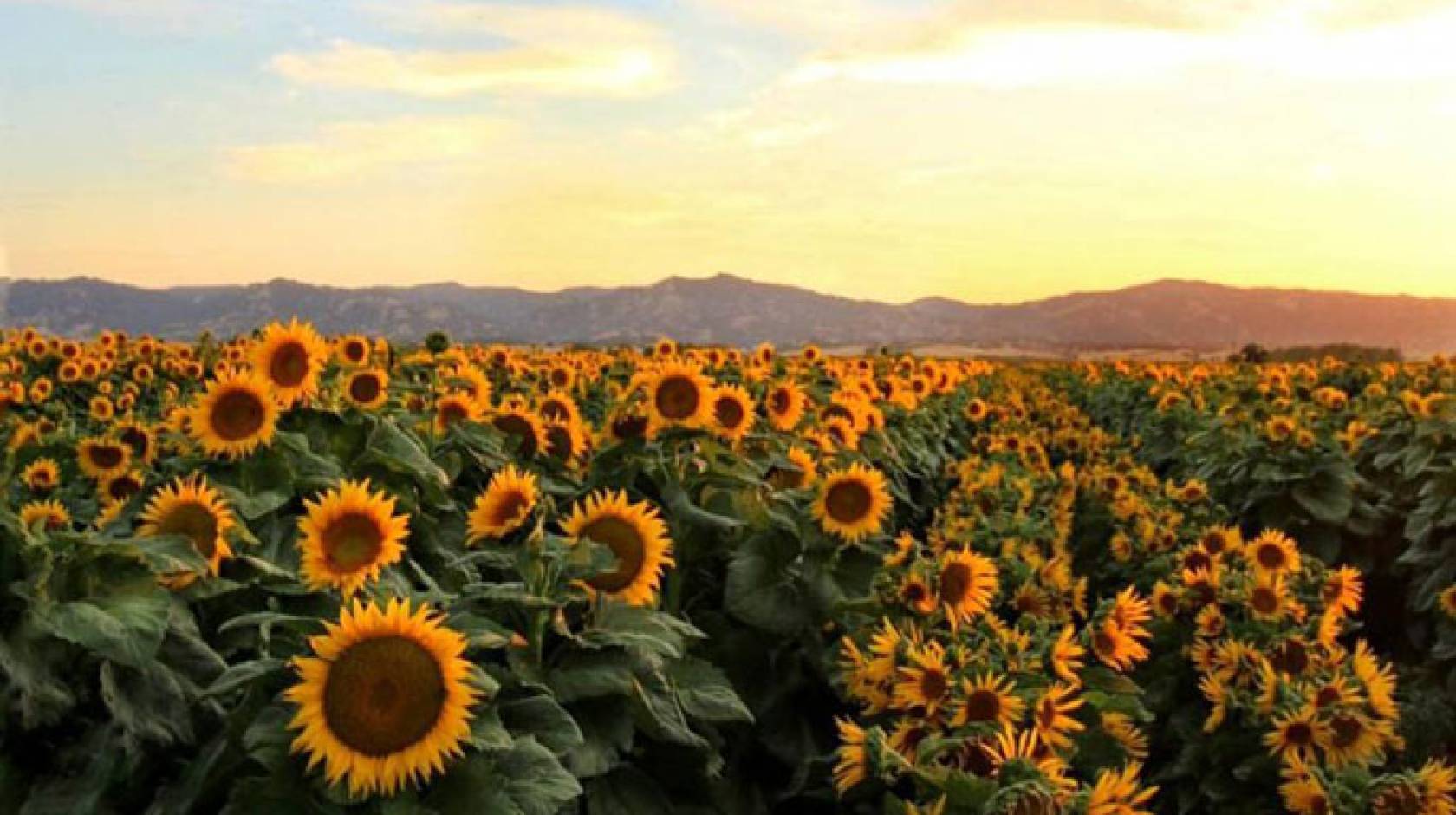This photo captures a serene scene of a commercial sunflower field stretching into the distance. The foreground is dominated by rows of sunflowers, their vibrant yellow petals encircling large, dark brown centers. The sunflowers are in various growth stages and heights, with some having prominent green leaves and stems. The meticulously arranged rows of sunflowers create a rhythmic pattern that draws the eye towards the center of the image. In the bottom left, particularly large sunflowers stand out, while smaller ones are scattered to their right. Beyond the field, a mountain range with its low-lying, slightly pointed hills extends from left to right. The sky above is a blend of golden hues and light blue, pierced by thin clouds, suggesting either dawn or dusk, adding a peaceful backdrop to the vibrant sunflower expanse.